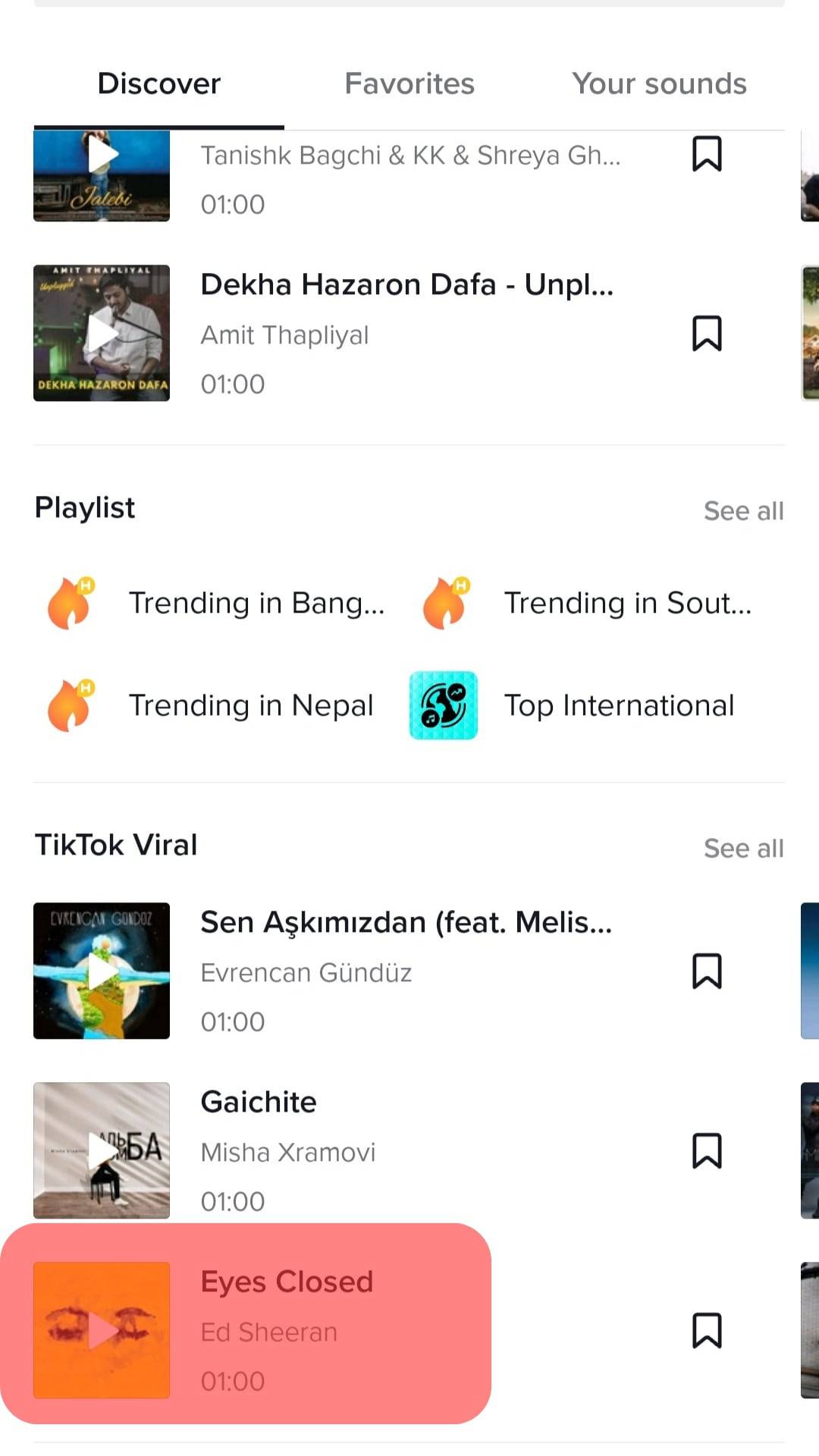### Image Description: Audio App Interface 
This image appears to be a screenshot of a cell phone displaying an audio app interface. The image itself is approximately two and a half times taller than it is wide. At the very top of the interface, there are three navigation tabs: 
1. **Discover** - The currently selected tab, highlighted in black.
2. **Favorites** - Grayed out, indicating it is not selected.
3. **Your Sounds** - Also grayed out, indicating it is not selected.

Beneath these tabs, the first section displays two albums on the left-hand side, both written in gray: "Tanishq Bagchi" and "KK Shreya GH," with an ellipsis ("...") suggesting there is more text.

Below this, another album is named "Deka Ke Sara Rang Dafa," also followed by an ellipsis.

Further down, there’s a section titled **Playlists** with several categories:
1. **Trending in Bangkok** - Indicated by a fire icon to the left.
2. **Trending in South...** - Again marked with a fire icon but the text is truncated.
3. **Trending in Nepal** - With another fire icon, positioned in the bottom left.
4. **Top International** - Marked with a teal icon, located in the bottom right of this section.

The bottom 40% of the screen is dedicated to another section, headed by **TikTok Viral**. This section displays three albums with the third one on the bottom right being highlighted by an overlay of a light red box, indicating it may be a popular or recommended selection.

This detailed description captures the various elements of the interface, providing a clear and thorough understanding of the image.